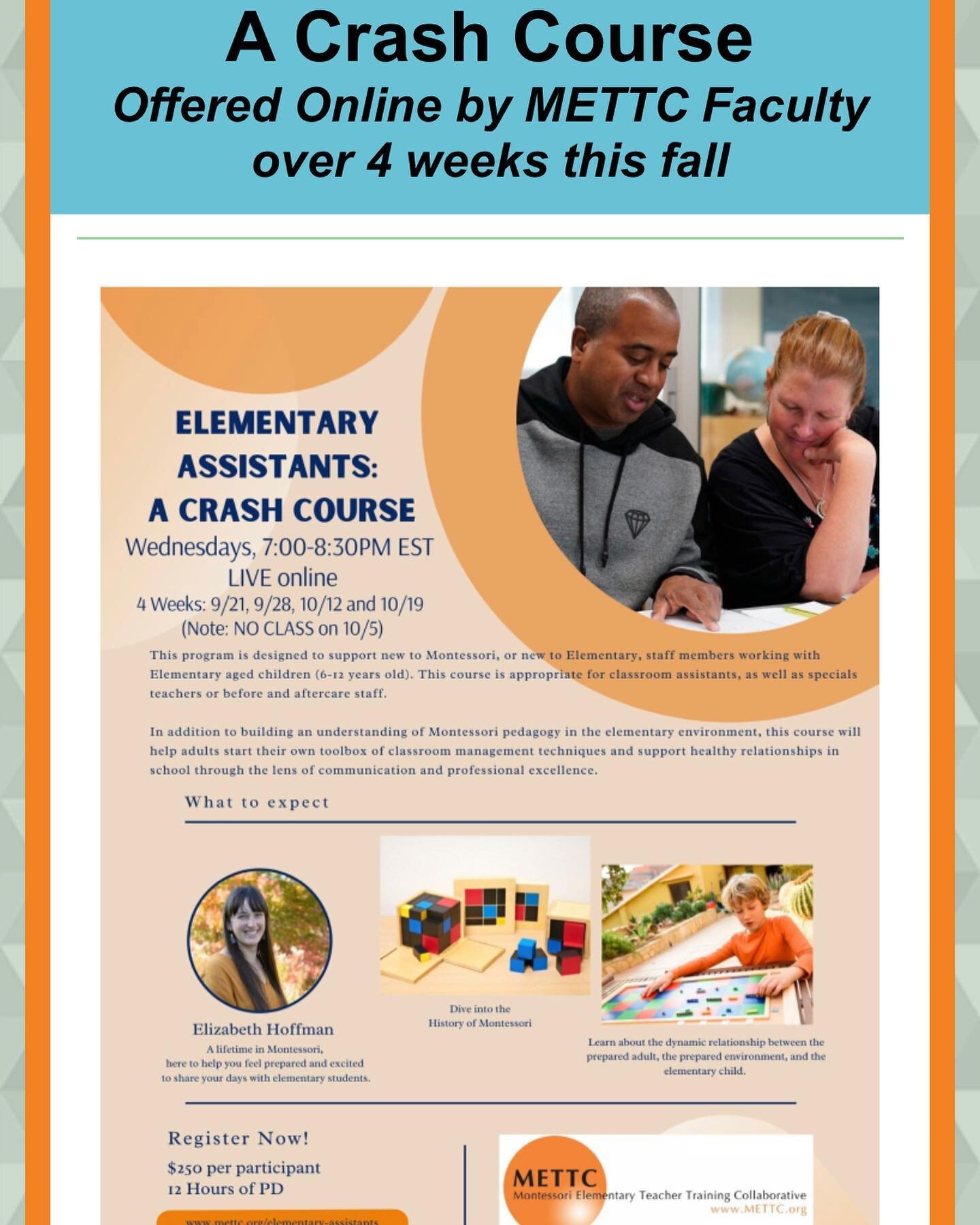This vertically oriented poster is a detailed advertisement for an online crash course offered by METTC faculty over four weeks this fall. It features a light blue horizontal banner at the top with black lettering that reads, "A crash course offered online by METTC faculty over four weeks this fall." Below this banner, the main content is presented against a white background and includes a pink rectangle with blue letters announcing, "Elementary Assistance: A Crash Course."

The poster is bordered on the left and right by light gray geometric shapes and additional vertical orange stripes. The course details are comprehensive: it is designed for new Montessori or new elementary staff members working with children aged 6 to 12 and will be conducted live online on Wednesdays from 7 to 8:30 p.m. EST across four weeks (Sept. 21, 28, Oct. 12, and Oct. 9, with no class on Oct. 5).

Costing $250 per participant, the program offers 12 hours of professional development and aims to support classroom assistants and special teachers in developing a toolbox of classroom management techniques. It emphasizes building an understanding of Montessori pedagogy and fostering healthy relationships through effective communication and professional excellence.

The poster also features a photograph of a diverse group of learners engaged in the course. Registration information and additional details, such as METTC's full name (Montessori Elementary Teacher Training Collaborative) and their website (www.METTC.org), are provided at the bottom. The course will be conducted by Elizabeth Hoffman, a seasoned professional with extensive experience in the Montessori educational system.